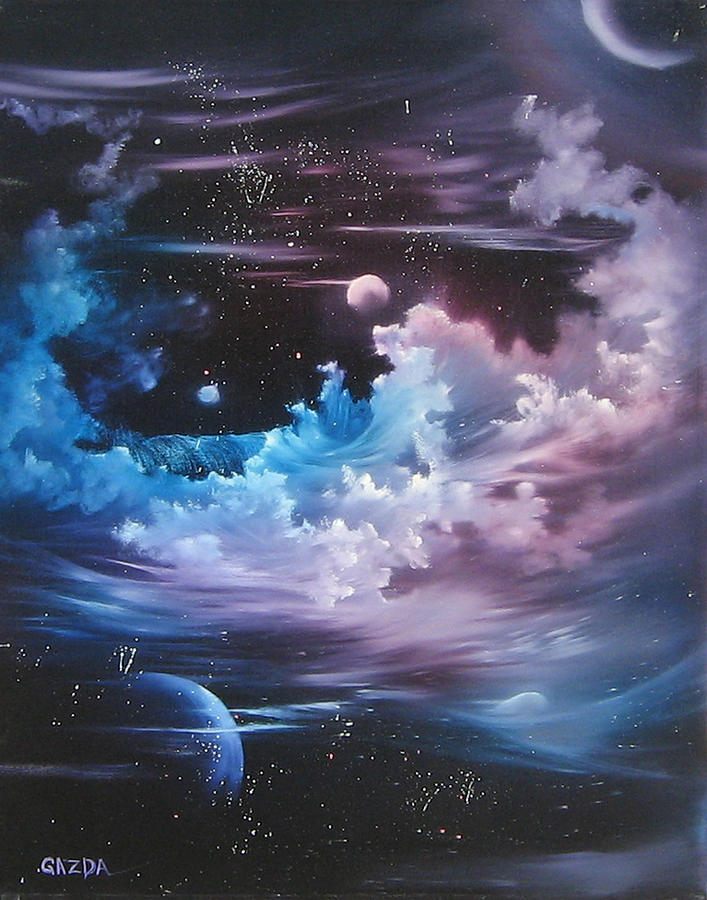This image is a highly detailed color illustration or computer-generated space art, portraying an imaginative interpretation of various celestial bodies against a vast, dark expanse. The majority of the background is a deep black, speckled with numerous star-like pinpoints, reminiscent of scattered paint splatters. 

Dominating the composition is a central bright sphere, perhaps a small white planet or moon, set slightly above the middle. Surrounding this celestial body are swirling clouds, colored in hues of blue, white, and purple, giving the impression of water waves turning into atmospheric phenomena. In the upper left corner, partially cut off, is another sphere with a distinctive white illumination along its edge, suggesting a glowing effect.

In the lower left corner, a larger planet with blue and dark hues is visible, partly shrouded in shadow and possibly representing Earth or a similar exoplanet. This planet is surrounded by more clouds, including a formation that looks like a wave crashing, with white caps blending into the clouds.

Adding a personal touch, the signature "Gaza" is prominently displayed in the lower left corner, marking the artist’s attribution. Overall, the illustration captures a vivid, imaginative view of space, blending elements of fantasy and cosmic grandeur.